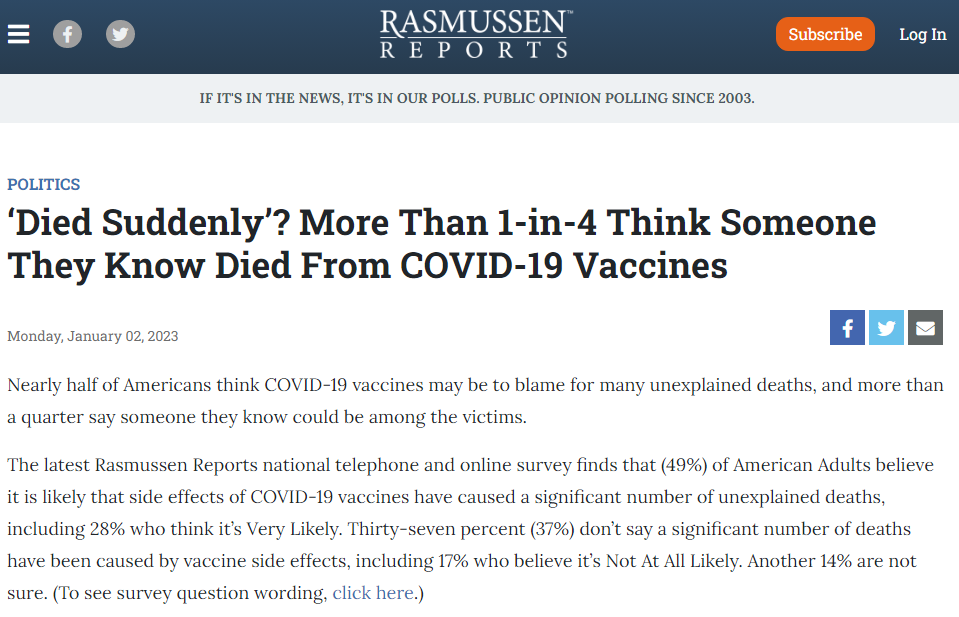This screenshot captures a detailed view of a website called Remuson Reports. The top navigation bar is rendered in a navy blue hue and features three horizontal bars on the left side, indicating a menu. Adjacent to these bars are two gray circles displaying icons for social media platforms, Facebook and Twitter. The website’s name, “Remuson Reports,” is prominently displayed in white text. To the right, there is an orange button labeled "Subscribe," also in white text.

Beneath the navigation bar lies a gray section, containing the tagline: "If it’s in the news, it’s in our polls - Public opinions polling since 2003." Below this tagline, the section headings are organized, starting with "Politics," written in blue text. The headline of the featured article reads, "Died Suddenly: More Than One in Four Thinks Someone They Know Died of COVID," dated Monday, January 2nd, 2023. Following the headline, the article content is presented, accompanied by options for sharing on various platforms.